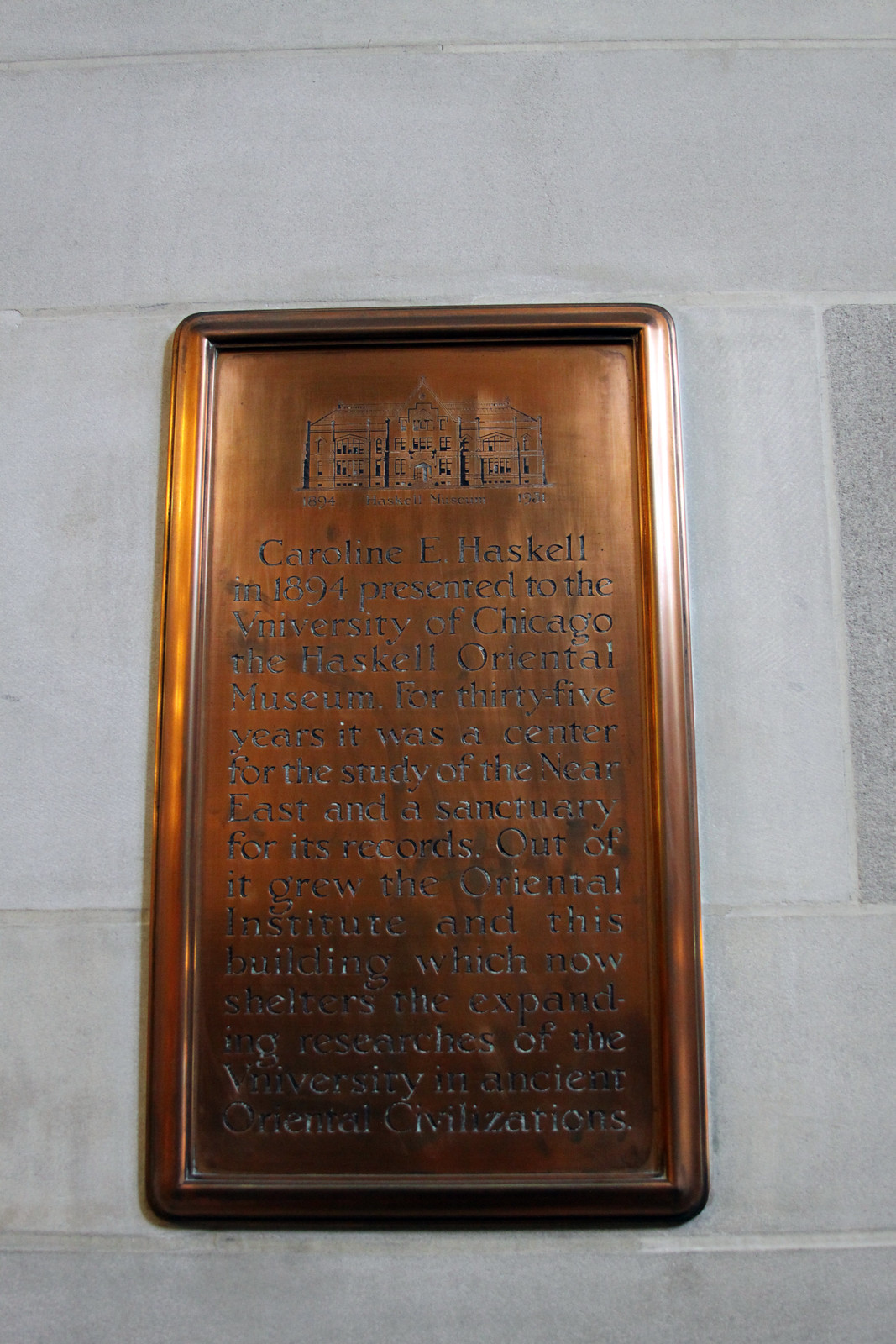The image features a vertically rectangular bronze plaque mounted on an off-gray white brick or granite wall. The plaque, encased in bronze and shining brightly, reflects a significant amount of light, making the details somewhat difficult to discern. At the top of the plaque, there is an engraved image of a building that appears to have three sections, resembling a mansion or a series of houses. Below the engraved image is text, reading: "Caroline E. Haskell, in 1894 presented to the University of Chicago, the Haskell Oriental Museum. For 35 years, it was a center for the study of the Near East and a sanctuary for its records. Out of it grew the Oriental Institute and this building which now shelters the expanding researches of the University in ancient oriental civilizations." The border of the plaque is raised, the text is etched in black, and despite some discoloration at the bottom, the top of the plaque appears almost brand new.